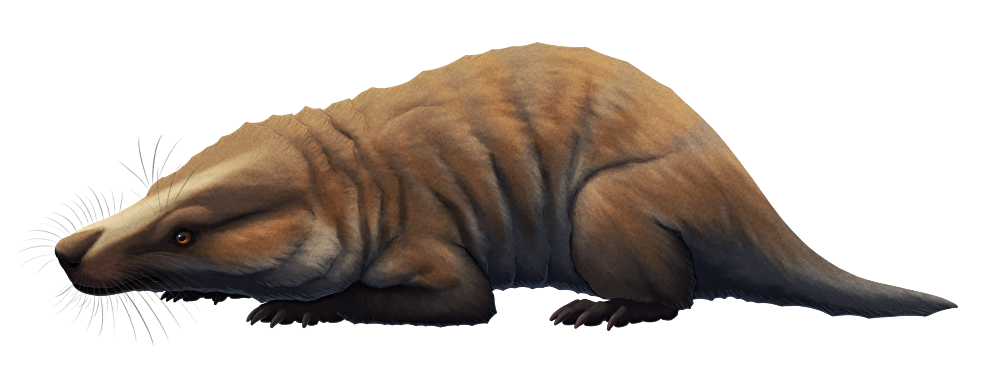The image depicts a digitally animated, detailed drawing of a small, brown animal resembling a combination of a badger, gopher, and raccoon. It is set against a white background. The creature, oriented to the left, features short fur, a semi-pointy, elongated snout, and noticeable whiskers. Its distinguishing characteristic is a white streak running from its nose up between the eyes, contrasting its predominantly brown fur. The animal is crouched down on its belly with its four legs tucked underneath, appearing as if it is ready to pounce or is hiding. Its short, broad tail and small paws with claws add to its distinctive appearance.